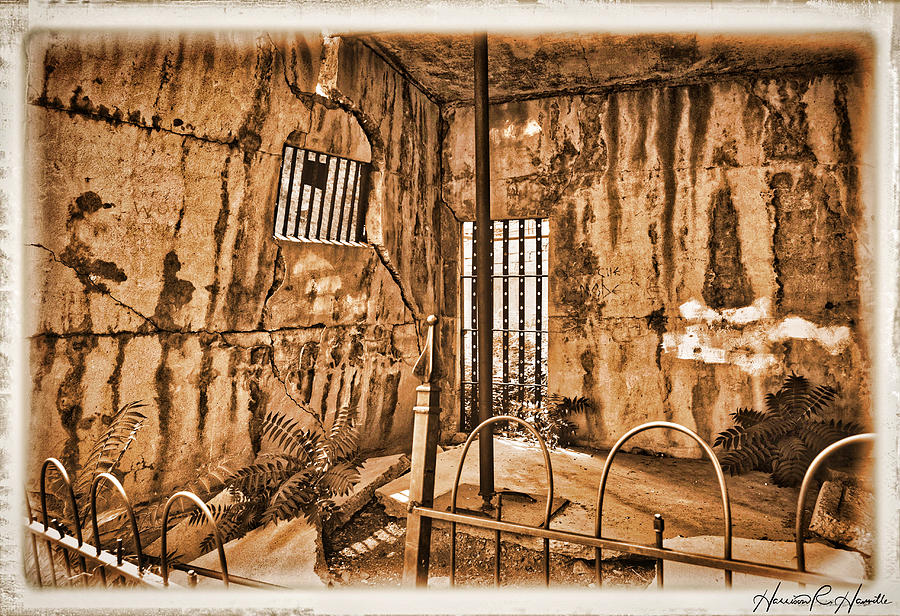This detailed painting depicts an abandoned and dilapidated jungle jail cell, crafted from crumbling concrete blocks, bearing the marks of age with large cracks and discoloration. The floor, made of broken concrete, reveals resilient plants growing through its fissures. The front of the cell is exposed, cordoned off by a thin metal fence featuring looping designs at the top. Inside, on the left wall, a square, barred window allows a glimpse of the dense vegetation outside, while a barred doorway stands in the background on the opposite wall. A long, slender metal bar extends from the floor to the ceiling at the center of the scene, adding to the atmosphere of decay. The overall coloration of the walls has a light brown hue, marred by black stains and streaks, contributing to the antique and historical ambiance of the artwork.